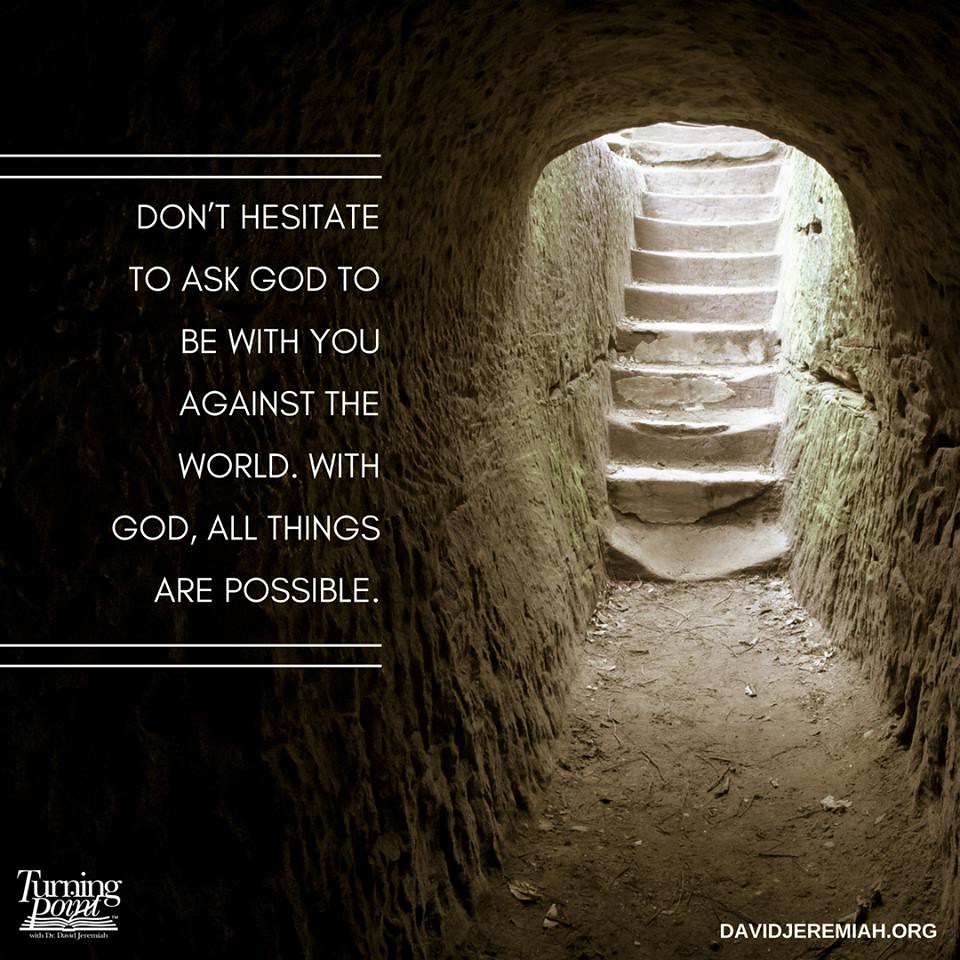The image depicts a dark, tunnel-like passageway with a dirt floor, scattered debris, and stone walls. At the top right, a set of rocky steps, illuminated by light from above, lead upward and out of the passageway. The text, "Don't hesitate to ask God to be with you against the world. With God, all things are possible," is prominently displayed on the left side of the image in white font, flanked by horizontal white bars above and below. The bottom left corner features the Turning Point logo alongside a graphic of a book, while the bottom right corner displays the website, DavidJeremiah.org, also in white. The overall composition and elements make the image appear as a motivational religious poster, accentuated by a palette of black, white, gray, brown, and tan.